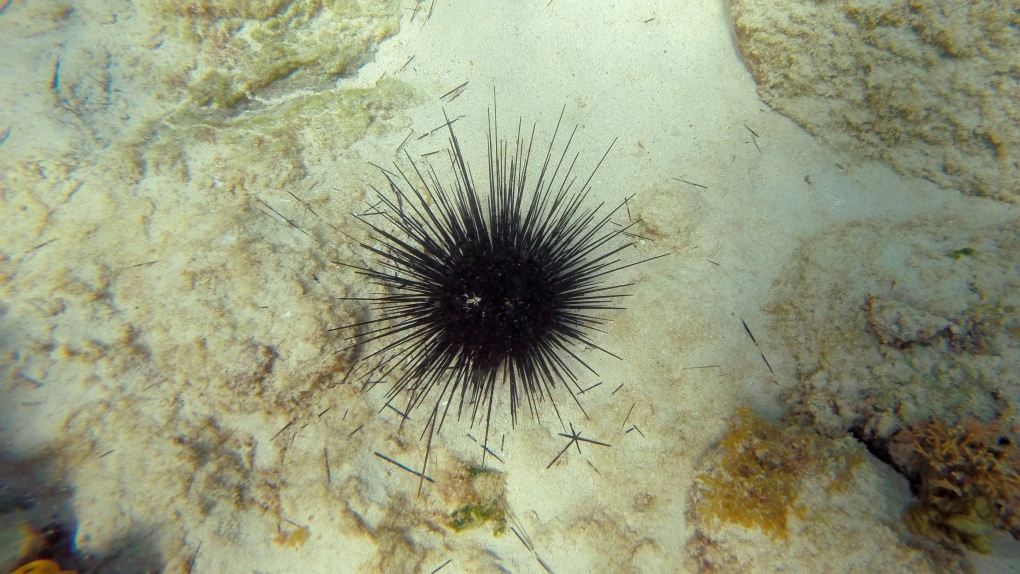This underwater color photograph captures a black sea urchin with long, needle-like spines centrally positioned on a sandy, beige sea floor. The spines of the urchin are prominently scattered around it, suggesting some have detached. The surrounding area is dotted with bumpy rocks and patches of coral displaying muted tones of orange, brown, and green, enhancing the natural, subdued color palette of the underwater scene. The absence of any people, other animals, man-made structures, or text emphasizes the sea urchin as the sole focal point of the image. The photograph, wider than it is tall, offers a serene glimpse into this isolated, coral reef environment.